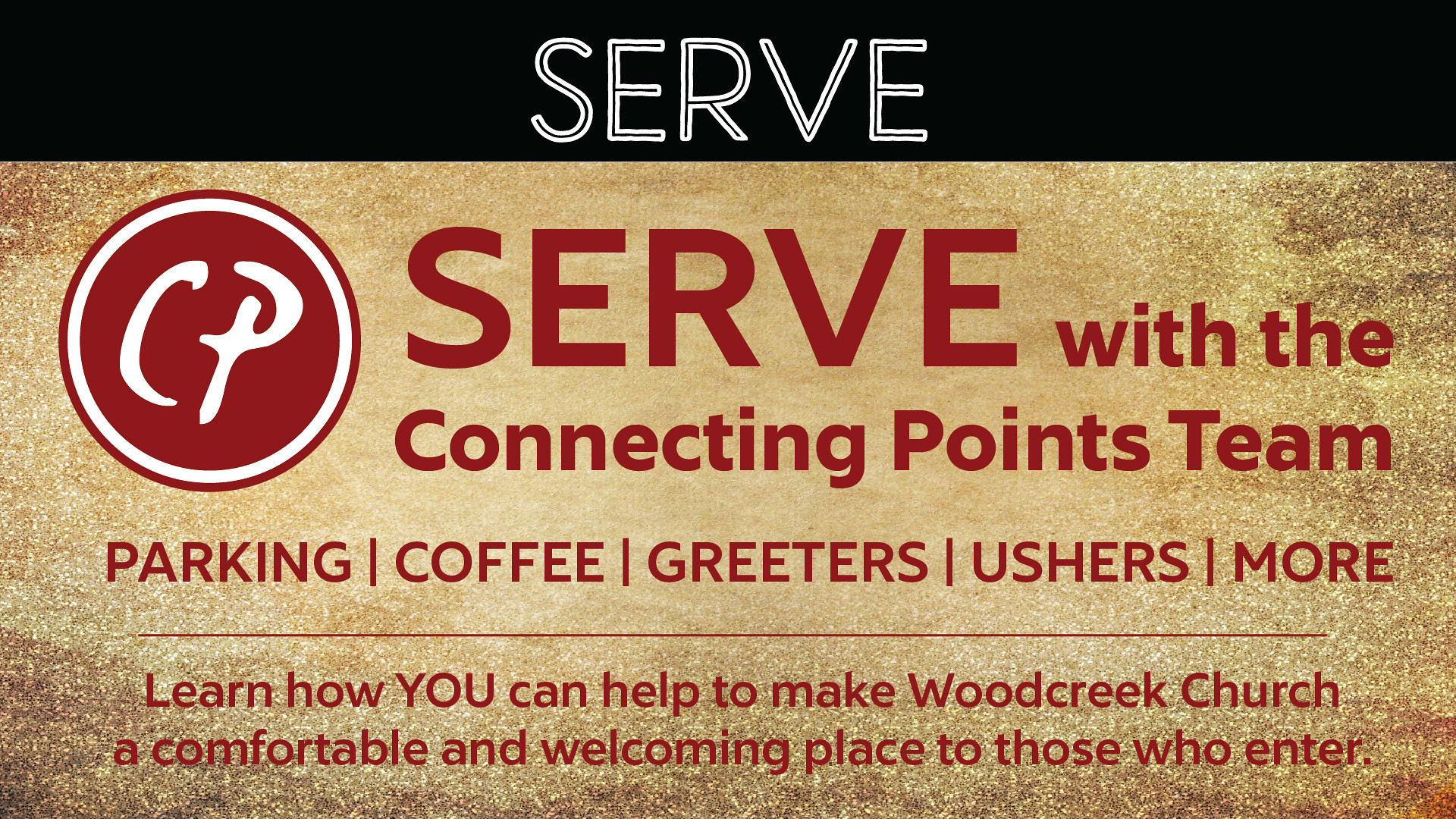The image appears to be an advertisement or promotional material for volunteering with the Connecting Points team at Wood Creek Church. It features a gold background with red, black, and white lettering. The text prominently says "Serve" at the top, followed by an invitation to "serve with the Connecting Points team." Key roles mentioned include parking, coffee, greeters, and ushers, listed in bold red text. Additionally, the image emphasizes the message: "Learn how you can help make Wood Creek Church a comfortable and welcoming place for others." On the left side, the letters "CP" are enclosed in a circle. The background primarily consists of black, but there are areas with a "scratching" effect that make some text more challenging to read due to varying colors and clarity.